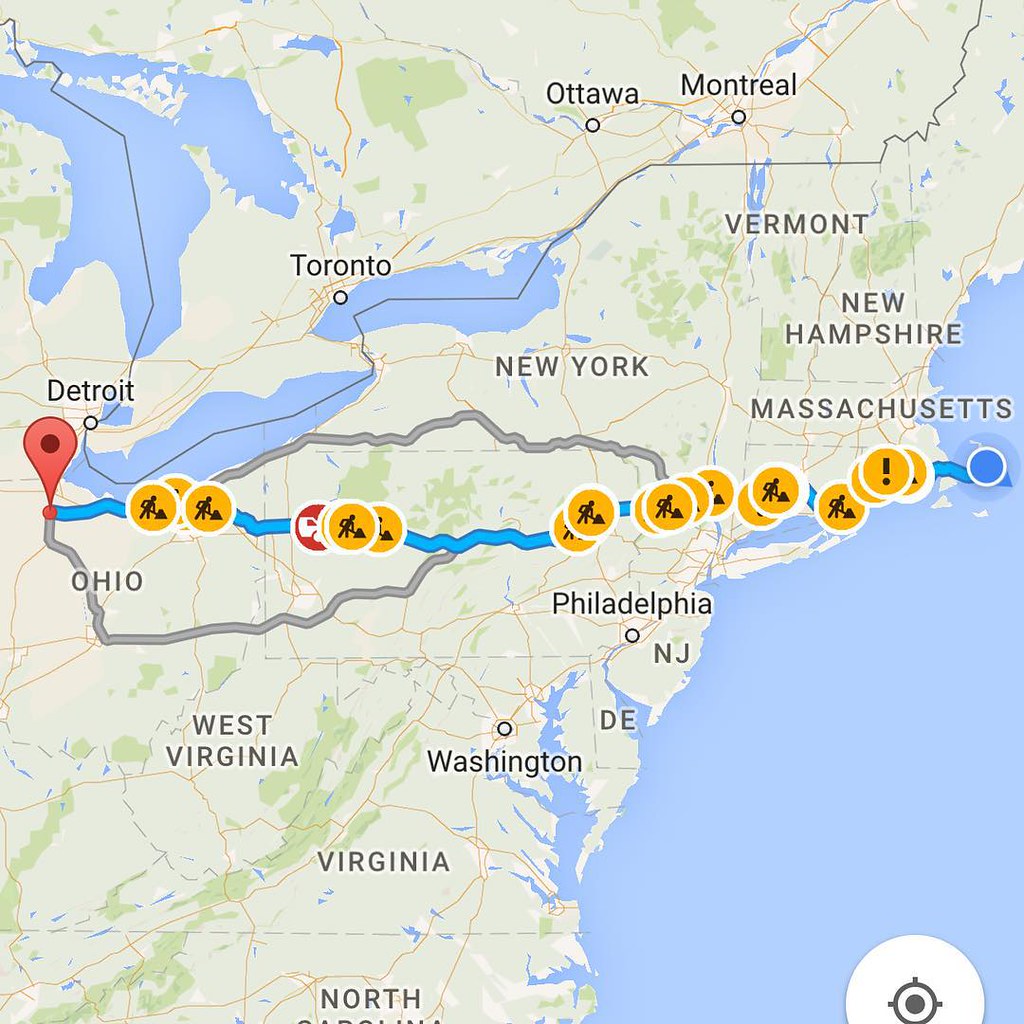This image depicts a detailed map of the northeastern United States and parts of Canada, primarily focusing on a route from western Ohio to a specific location off the coast of Massachusetts, likely an island. The map features three distinct routes. The main route is highlighted in blue, indicating areas affected by construction and traffic jams due to an accident. Two alternative routes are marked in gray. The map is annotated with state names, major city names, including U.S. cities, and some Canadian cities such as Toronto, Ottawa, and Montreal.